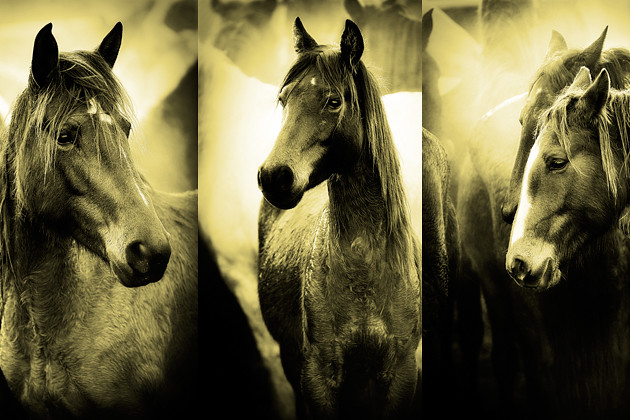The photograph features a black and white triptych of horses, each panel offering a different, detailed perspective. The first image on the left captures a left-side view of a dark grayish horse with perked, pointy ears and a distinctive white star on its forehead. The horse's forelock cascades down over its eyes, adding character to its expressive face. The middle panel showcases a younger grayish horse, viewed head-on but gazing to the right. It too has forward-facing ears and a small white dot on its forehead. In the final panel on the right, the heads of two horses are depicted side by side. The prominent horse displays a striking white stripe running down its face, its ears slightly back and a thick mane flowing. The second horse’s head is partially obscured behind the first, adding a sense of depth. All three images share a captivating monochrome palette, accented by subtle hints of yellow that enhance the visual interest and coherence of the triptych.